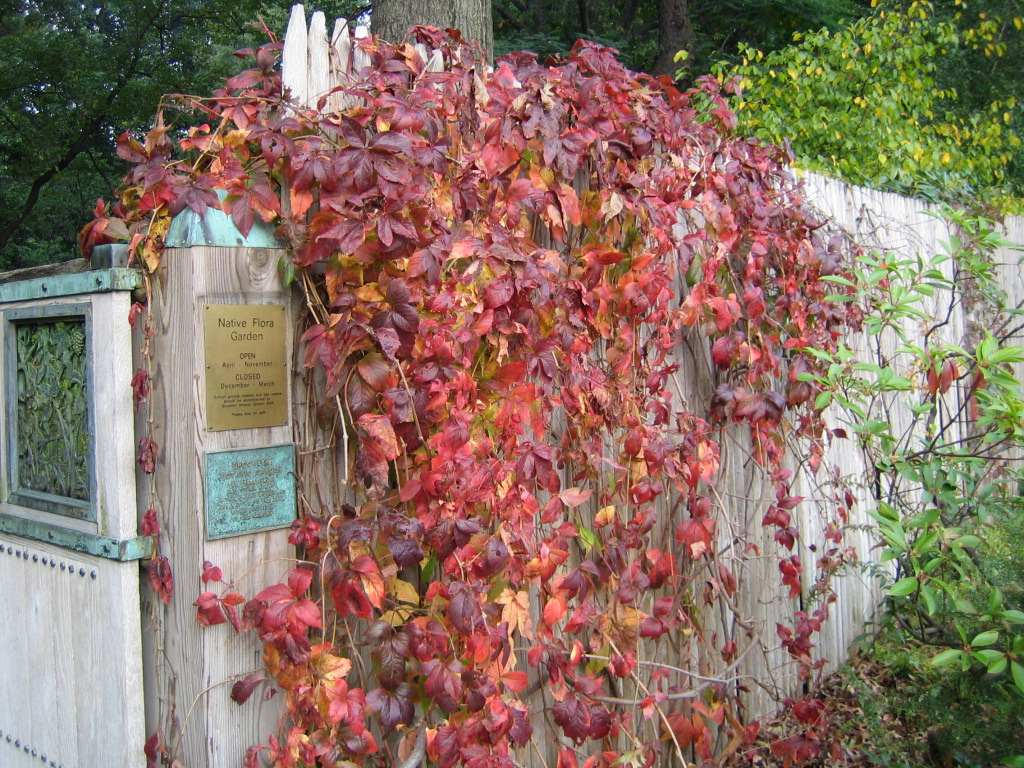The photograph captures an outdoor scene of a heavily overgrown white picket fence that appears to serve as an entrance to a floral garden. The fence stretches diagonally from left to right in the image, with the left side of the fence being closest to the camera and the right side receding into the background. Densely packed green foliage can be seen in the background, along with additional greenery surrounding the scene.

The fence is predominantly overgrown with a vine that sports dark reddish-purple leaves, indicating the photo was likely taken during the fall season as the leaves are changing colors. These vibrant leaves cover the front portion of the fence, with some overhanging the top and trailing behind.

Significantly, a wooden fence post is located on the left side of the photograph. This post holds two plaques: the top one being gold with black writing that states, "Native Floral Garden open April to November," and the lower one being a painted blue square with text too small to read clearly. To the left of the post, there's a partial view of a white painted wooden gate that appears clean and less affected by the overgrowth, suggesting it serves as an entrance to the garden. The presence of green trees in the background adds to the depth and lushness of the scene.